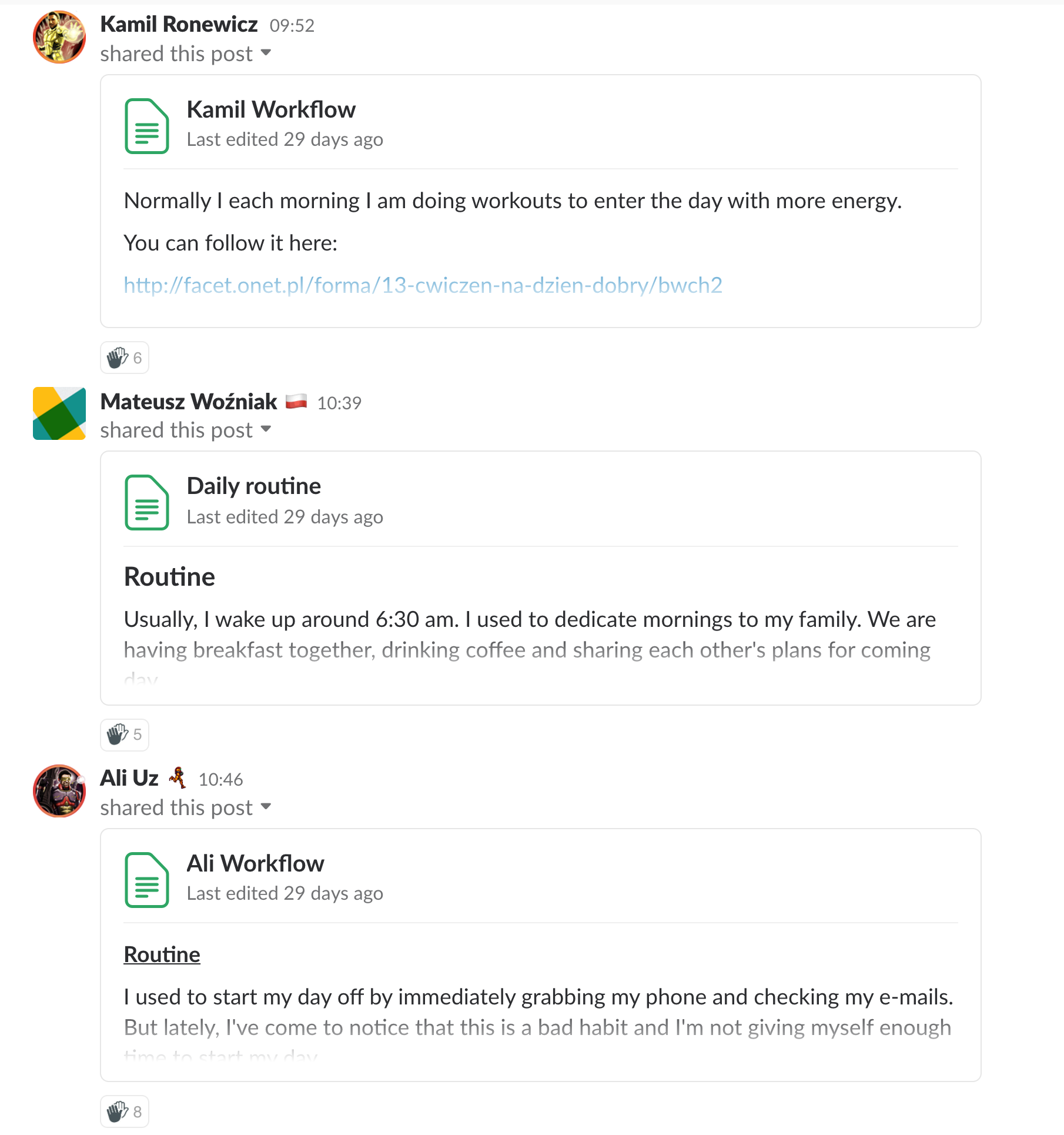This image captures a snapshot of a social media-style webpage dedicated to job-related postings. The interface has a clean, minimalist design with a completely white background and black or dark gray text for high readability.

At the top of the page, there's a post from Camille Ronewicz. The detailed text reads: "Camille Workflow." This post was last edited 29 days ago. Immediately below is another post from Matus Wozniak, which mentions that Matus shared a "Daily Routine" post. This entry was also last edited 29 days ago.

Following Matus's post, there's a contribution by Allie Uz, indicating that Allie shared another post. Beneath this is a more specific post titled "Allie Workflow," similarly last edited 29 days ago. 

The collective theme of these postings suggests that this is a collaborative workspace where employees share their daily routines and workflows for others to download and reference. This feature likely facilitates a better understanding of each person's workflow and promotes transparency and efficiency within the team or organization.